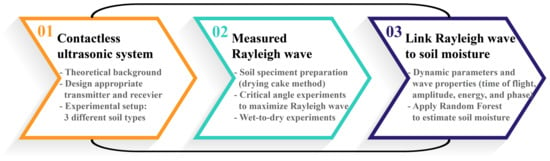The image is a flowchart consisting of three sequential sections, each shaped like an arrow and labeled numerically. The first arrow, outlined in orange and labeled "01," reads "Contactless Ultrasonic System." It contains details on theoretical background, designing appropriate transmitters and receivers, experimental setup, and three different soil types. The second arrow, in teal blue and labeled "02," is titled "Measured Rayleigh Wave" and elaborates on soil specimen preparation, the drying cake method, critical angle experiments to optimize Rayleigh wave generation, and wet-to-dry experiments. The third arrow, outlined in dark purple and labeled "03," is titled "Link Rayleigh Wave to Soil Moisture," and includes factors such as dynamic parameters and wave properties, time of flight, amplitude, energy, phase, and the application of random force to estimate soil moisture. The entire diagram is contained within an oblong green line, presenting a comprehensive process from initial contactless ultrasonic setup to the measurement and application of Rayleigh waves for soil moisture analysis.